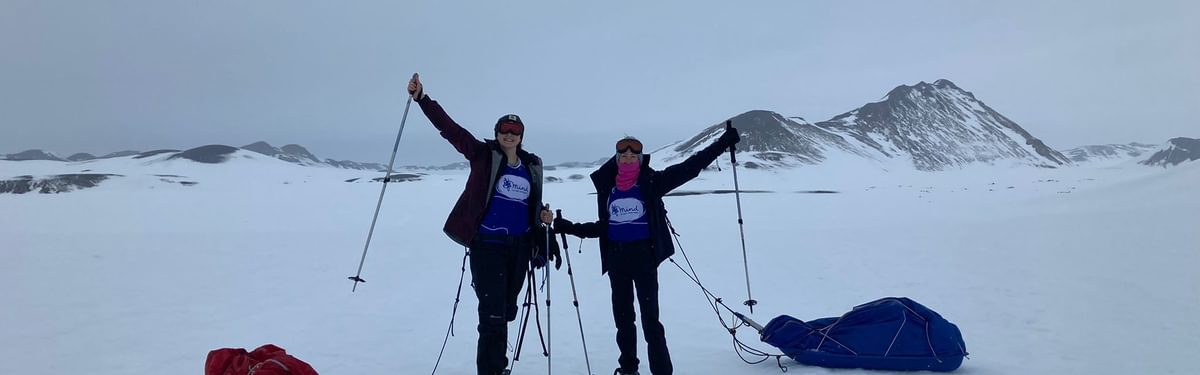This detailed color photograph, oriented in landscape, captures two individuals standing together at the center of a snow-covered field. Both individuals are dressed in dark, unzipped jackets, black snow pants, and matching blue vests with white placards featuring illegible text. The taller person, possibly a woman, and the smaller individual both wear goggles, hats, and face masks, emphasizing their preparedness for cold conditions. They stand close to one another, facing the camera, with each raising an arm to hold a ski pole aloft while their other hands are braced into the snow with ski poles. The backdrop is a dramatic panorama of hazy, snow-covered hills under a dark grey, fog-laden sky, enhancing the sense of isolation and adventure. Two colorful parachutes or tent-like objects, one blue and one red, are visible behind them, adding vibrant accents to the predominantly monochromatic landscape. To the right of the taller individual is a sled-type object, covered and wrapped with ropes, suggesting they are on a significant excursion or perhaps celebrating a momentous achievement atop the mountain.